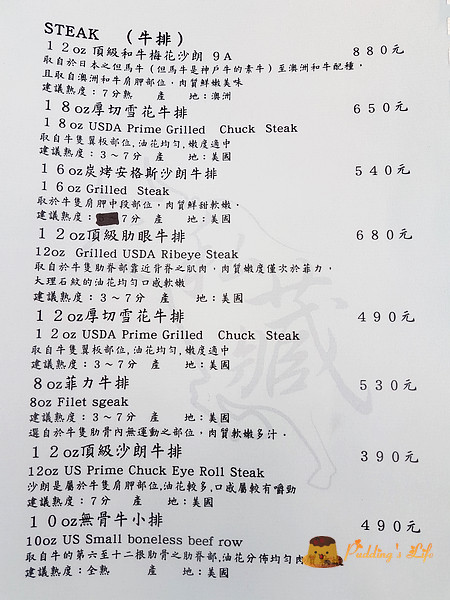The photograph depicts the menu of an Asian restaurant, predominantly written in what appears to be Mandarin Chinese. The menu features English translations alongside the original text for a selection of items. These English translations are situated towards the left side of the menu, with corresponding descriptions and translations in Mandarin Chinese. On the right side, a column displays the prices for each item, neatly aligned in a vertical row. At the bottom of the menu, beneath the prices, a small cartoon character that resembles a dessert is illustrated. Adjacent to the character, yellow-orange text provides additional information. Notable menu items readable in English include:

- Steak, 8 ounces
- One 8-ounce USDA prime grilled chuck steak
- One 6-ounce grilled steak
- 12-ounce grilled USDA ribeye steak
- Filet steak

The majority of the menu, however, remains in Mandarin Chinese, adding to the authenticity and cultural ambiance of the establishment.